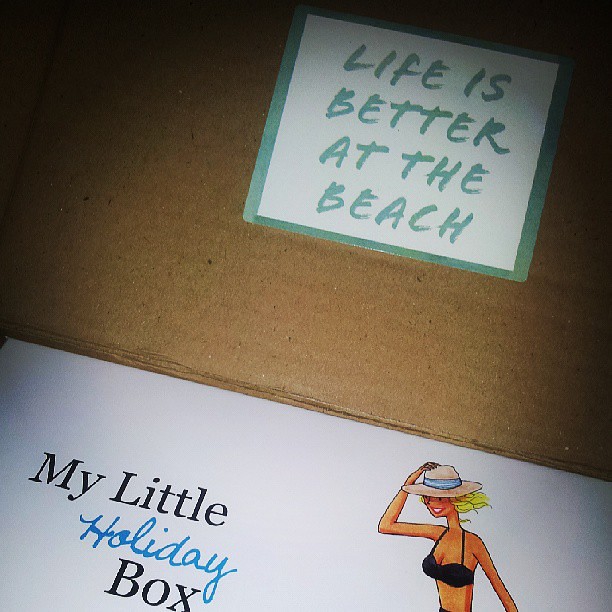The image is a detailed photograph of an open brown cardboard box. Inside the box, the top inner lid has a white sticker with a teal green border and text that reads "Life is better at the beach" in a neat, all-caps font. Below the open lid, there is a smaller white box situated inside the larger brown cardboard box. This white box is titled "My Little Holiday Box" with the word "Holiday" written in blue cursive and the rest in black Arial font. To the right of this text, there is a graphic, cartoon-like drawing of a woman in a retro-style black bikini and a sun hat, which she is holding against the wind. The woman has short blonde hair, and the overall design suggests a cheerful, beach-themed package.